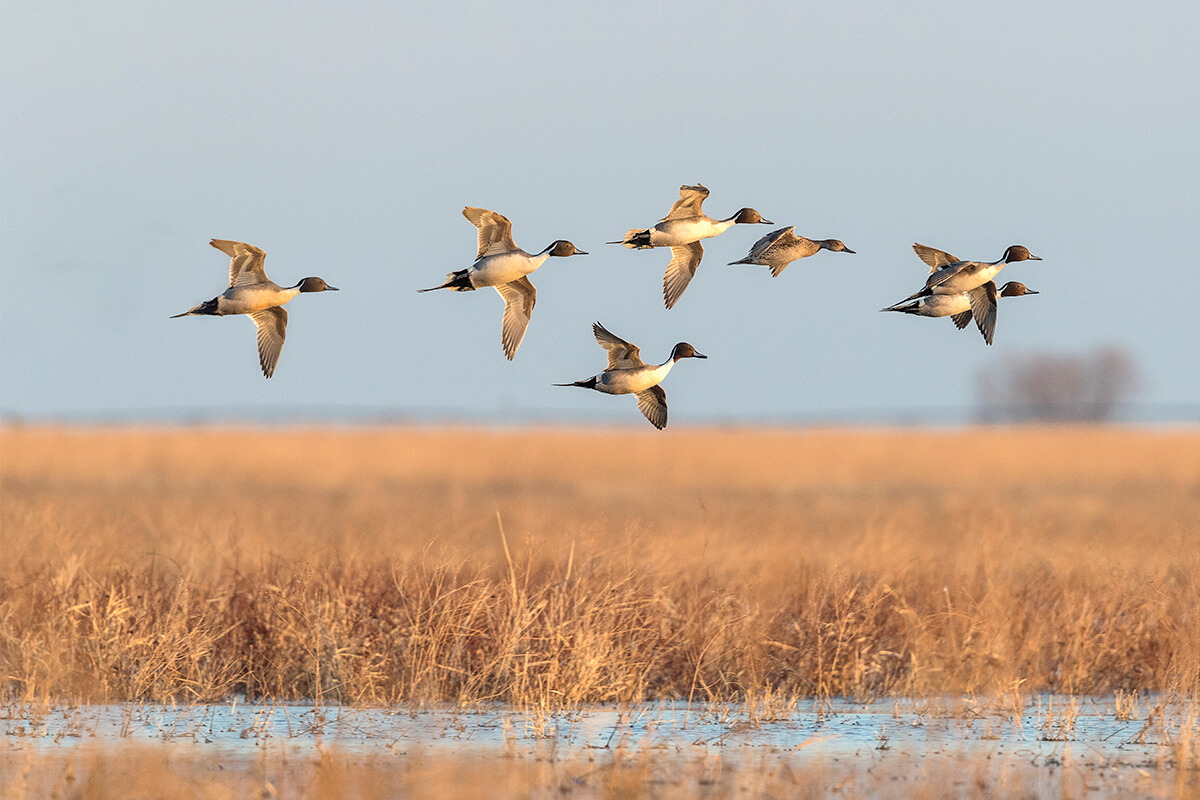The photograph captures a scene of seven birds, likely geese or ducks, flying with their wings outstretched over a expansive marshland. The landscape features dry, brown, marsh-like grass interspersed with patches of water. The birds, displaying a mix of white, gray, and brown colors with white bellies and brown heads, are sharply in focus as they glide toward the right side of the image. In contrast, the background is slightly blurred, including a distant, brown tree on the far right. The sky above is a muted bluish-gray, typical of an overcast day, adding to the serene, yet desolate atmospheric feel of the wetlands. The overall composition suggests the image was taken during daytime from an elevated perspective.